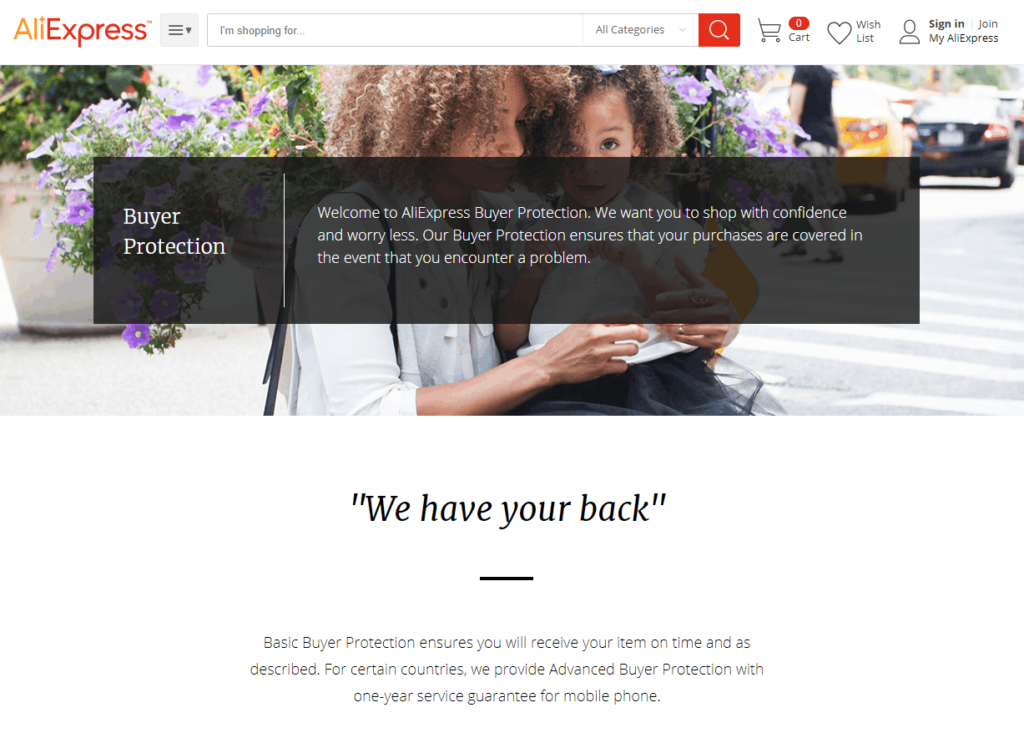This image is a detailed screenshot of the Aliexpress website, captured from a computer screen. The Aliexpress logo is prominently displayed at the top left corner in a gradient of orange and red hues. To the right of the logo are three horizontal lines accompanied by a heart icon, which likely represents the menu or favorite items. 

Centered on the top navigation bar is a search bar containing the placeholder text "I'm shopping for..." followed by an option to browse "all categories." To the right of the search bar, a red box featuring a white search icon invites users to perform searches. Adjacent to the search box is an icon of a shopping cart with the word "Cart" and the number zero inside a red oblong circle next to it, indicating an empty cart. Further along, a heart icon signifies a wish list feature, and an icon of a person followed by "Sign In" prompts users to access their accounts or join Aliexpress.

Dominating the center of the screen is a long picture depicting a woman with her child seated on her lap amidst a backdrop of flowers. In the background, a person walking and a few cars suggest light traffic or a casual street scene. 

Overlaying this image is a long rectangular bar that states "Buyer Protection." The text within the bar reads: "Welcome to Aliexpress Buyer Protection. We want you to shop with confidence and worry less. Our buyer protection ensures that your purchases are covered in the event that you encounter a problem." Just below this main header, in parentheses, it reassures users: "We have your back."

Beneath the image, it describes the terms of "Basic Buyer Protection," assuring that items will be received on time and as described. Additionally, for certain countries, Aliexpress offers "Advanced Buyer Protection," which includes a one-year service guarantee for mobile phones.